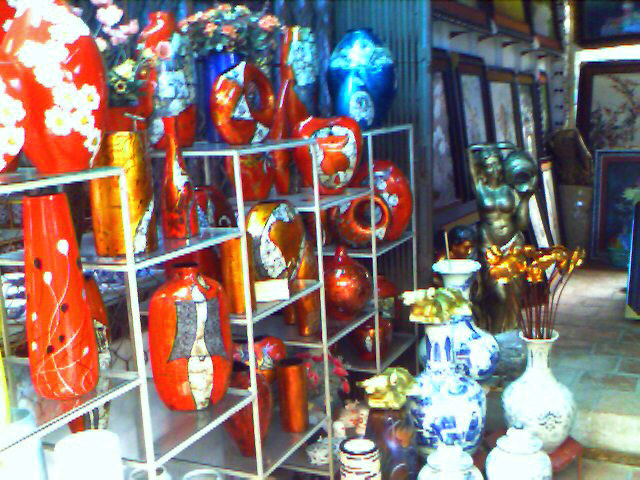A vibrant and eclectic display of vases is showcased in a possible antique store or designer showroom. The arrangement is on square-edged, multi-level metal and glass shelves with the majority of vases being a striking red adorned with a variety of designs, including animals, floral patterns, and avant-garde motifs resembling balloons on strings. Noteworthy pieces include a short, round red vase with blue and white geometric designs, a tall thin red vase with a black and white balloon decoration, and another slightly oval red vase featuring a gray square and white squiggle. Interspersed among these are larger blue vases positioned on the top shelf at the back. Below, a collection of white porcelain or china vases, some with floral arrangements, adds contrast. In the backdrop, there are multiple large framed portraits, murals, and pictures either hanging on the wall or standing on the floor. Adding to the artistic ambiance, a prominent statue of a mermaid, likely designed as a fountain piece, and a statue of a woman holding a vase, contribute to the overall visual appeal of this overexposed but colorful photographic capture.